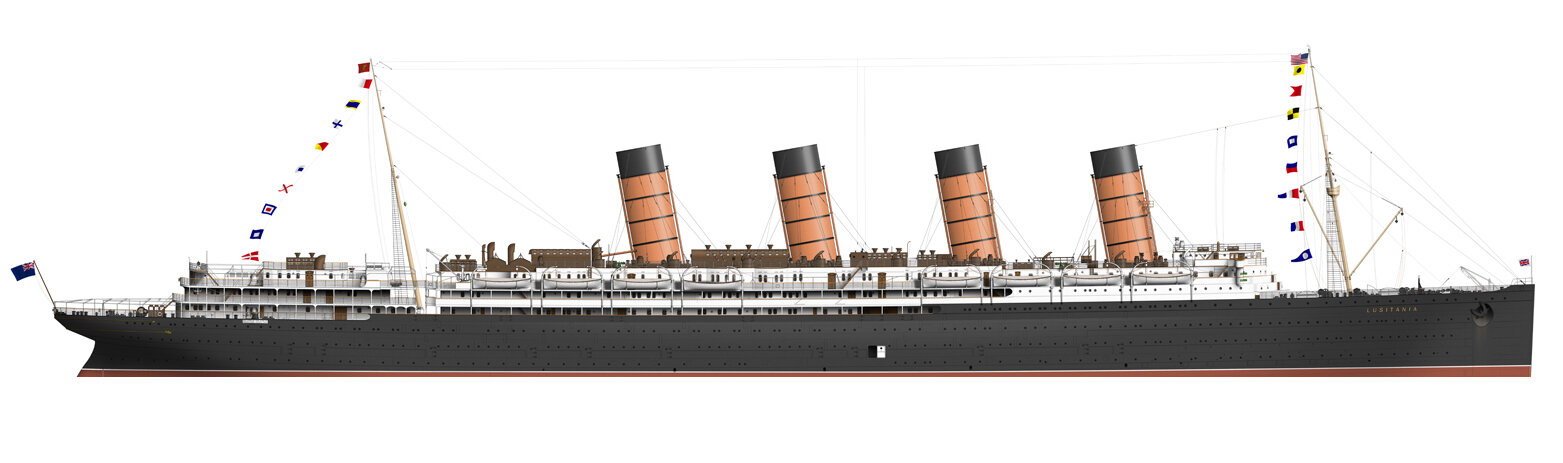This side view image depicts a meticulously crafted model of an early 1900s ocean liner, showcasing the vessel's classic and iconic design. The ship's black hull contrasts strikingly with the white decks above, which are punctuated by numerous windows that hint at the elegance within. Dominating the uppermost deck are the ship's distinctive smokestacks, which are slanted towards the left and feature a brown body with black tops. Both the fore and aft sections of the ship are adorned with poles from which various flags are suspended, cascading down towards the lower front and bottom decks, adding a touch of maritime authenticity. The model captures the impressive length of the ocean liner, conveying the grandeur and engineering marvel of early 20th-century maritime travel.